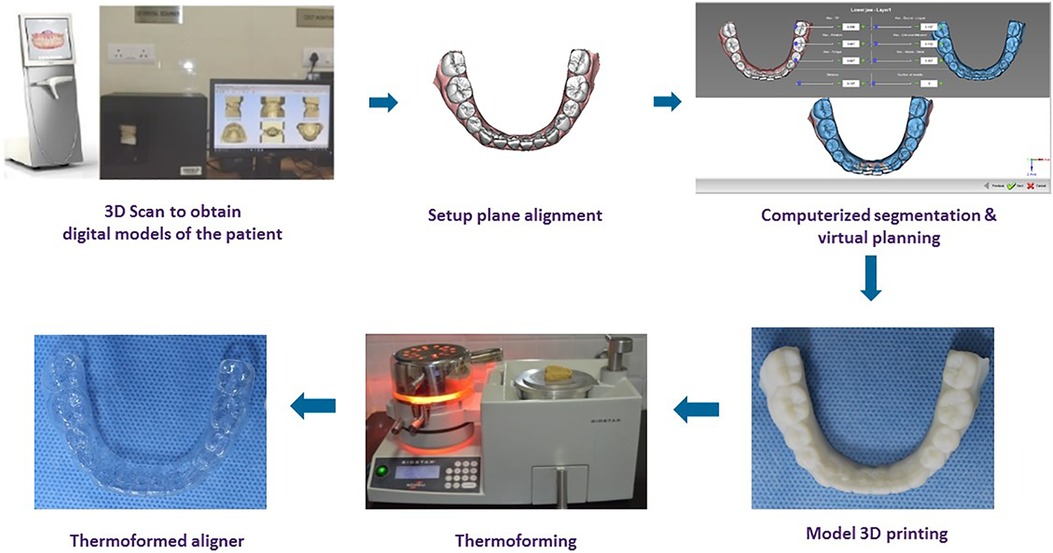The illustrated flow chart depicts a comprehensive six-step process for creating dental aligners, commonly used for teeth straightening like Invisalign. The first step involves a 3D scan to obtain digital models of the patient's teeth, highlighted by an image of a 3D scanner and a monitor displaying the scanned model. Next, the setup plane alignment is shown, featuring an image of the digital alignment of the teeth. The process then moves to computerized segmentation and virtual planning, breaking down the upper and lower plates through detailed diagrams and descriptions. This step is connected to the following steps with arrows. The fourth step, model 3D printing, displays a 3D-printed model of the teeth. In the next phase, thermoforming, a machine with a glowing red light molds the 3D printed model. Finally, the process concludes with the creation of a clear thermoformed aligner, ready for use in straightening the patient's teeth. The entire sequence visually demonstrates the meticulous and technologically advanced workflow in dental aligner production.